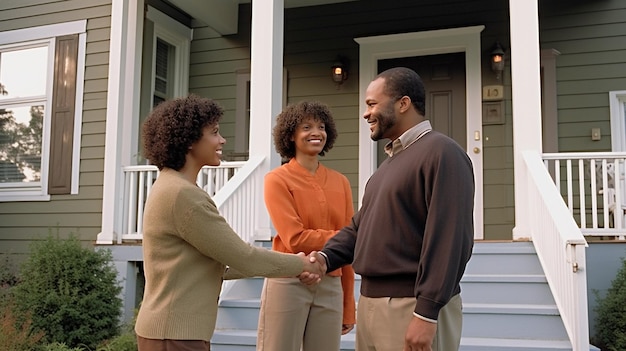In front of a newly built, middle-class home with light brown siding and white borders, three smiling African American individuals, two women and one man, pose for a photograph. The man, on the right, is dressed in a dark brown sweater over a buttoned-down shirt and tan slacks. He has a short beard and short hair. He is shaking hands with a woman on the left, who wears a beige sweater and brown pants. Standing between them is another woman, dressed in an orange long-sleeve shirt and beige pants, facing the man with her right arm extended, as if preparing to shake his hand next. Both women, who appear to be twins with their short, curly black hair and similar facial features, are smiling widely. The backdrop of the image includes gray steps leading to a front door flanked by lit porch lights, suggesting an advertisement for a real estate company.